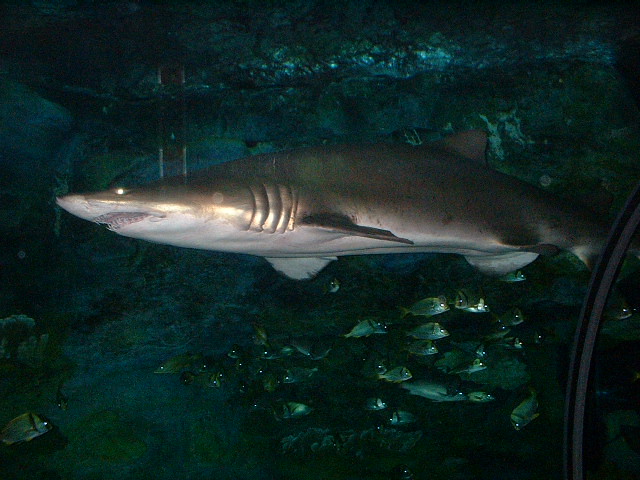The image depicts an underwater scene, likely taken in an aquarium or the ocean. The central focus is a large adult shark, shown in a side profile swimming to the left. Its features, including a triangular nose, slightly open mouth revealing teeth, glowing eyes, and distinct gills, are visible in detail. The shark's body is grey on the top and sides, with a white underside. Below the shark, a school of small oval-shaped fish swims in various directions. The background is dark and rocky with a teal tint, adding to the overall dim lighting of the scene. The colors in the image predominantly include black, grey, blue, green, and white, with no text present. Additionally, a black strip on the right side suggests the edge of a clear window, reinforcing the aquarium-like setting.